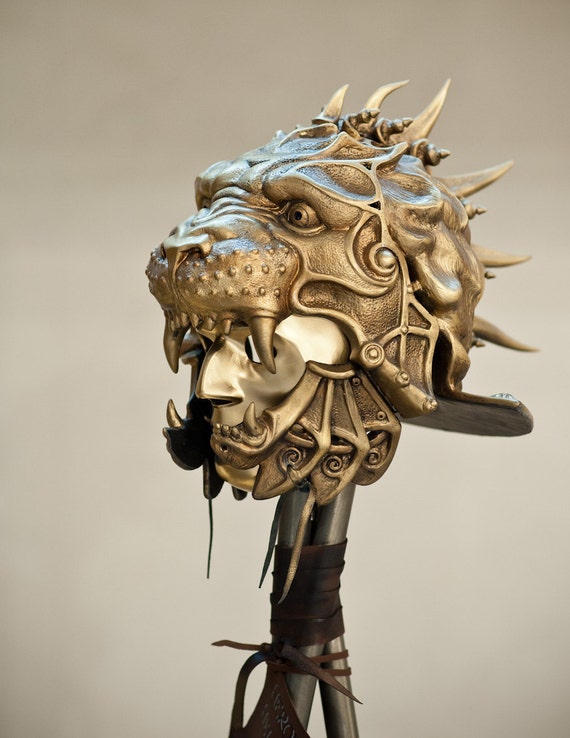The image depicts an intricate, bronze-colored historical helmet, designed with a two-tiered mask structure. The lower portion features the menacing face of an ogre or Lord of the Rings-style orc, complete with long bottom incisors. Above it, the top tier showcases the fierce visage of a tiger-like mythical creature, its mouth agape to reveal a human face within. This creature's design includes ferocious incisors along with spikes protruding from the back of its head, further adding to its mystical appearance. The helmet is mounted on an upright metal post, secured with leather straps, and it is displayed on a mannequin for a full profile view. The detailed craftsmanship and the combination of feral and humanoid elements suggest it was a ceremonial artifact or a part of ancient armor, reflecting both power and artistry.